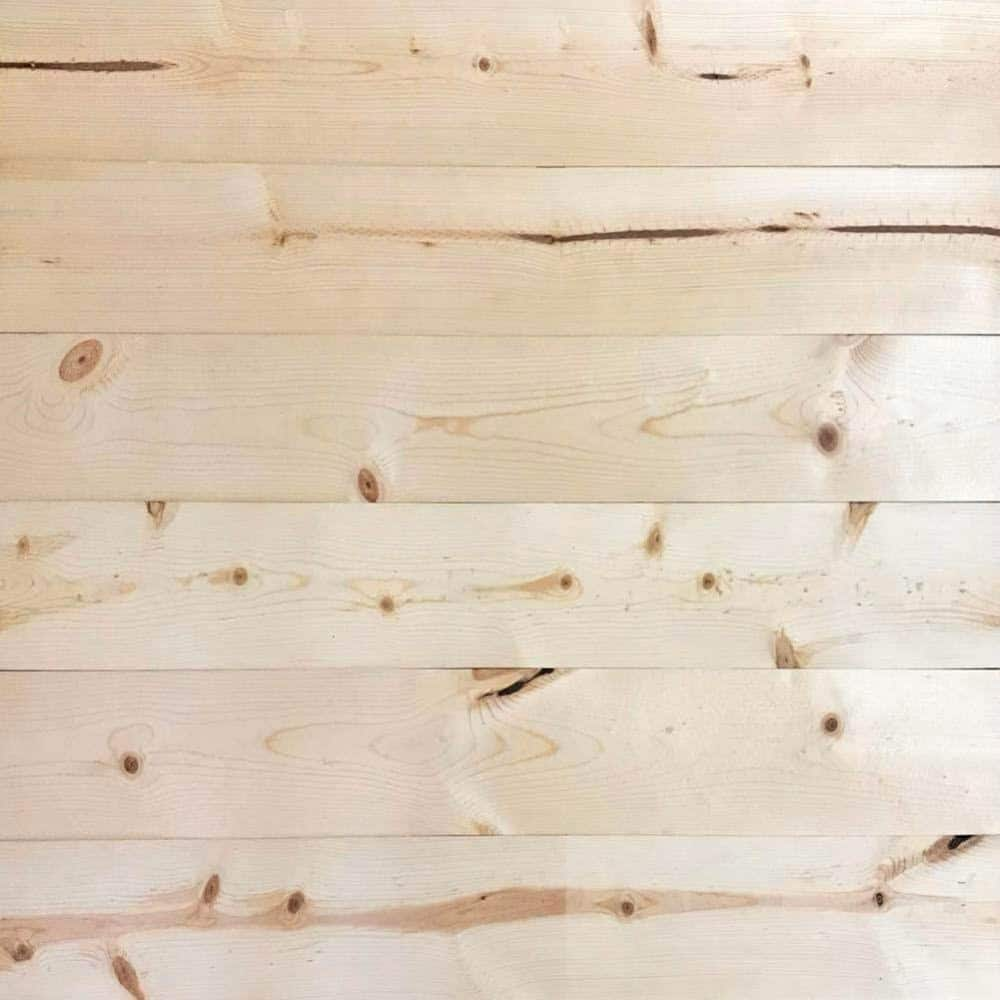The image depicts a photorealistic close-up view of light-colored wood paneling, likely pine, that makes up an entire wall or surface. The six horizontal wood planks dominate the image, characterized by their unfinished, unstained light tan or beige color with visible wood grain patterns. The grain includes some very dark brown streaks and numerous knots, some of which appear as oval blemishes, adding to the natural texture and imperfections of the wood. The photograph details the natural beauty and uniqueness of each plank, with no visible edges or nails, capturing the intricate details and subtle light reflections on the surface.